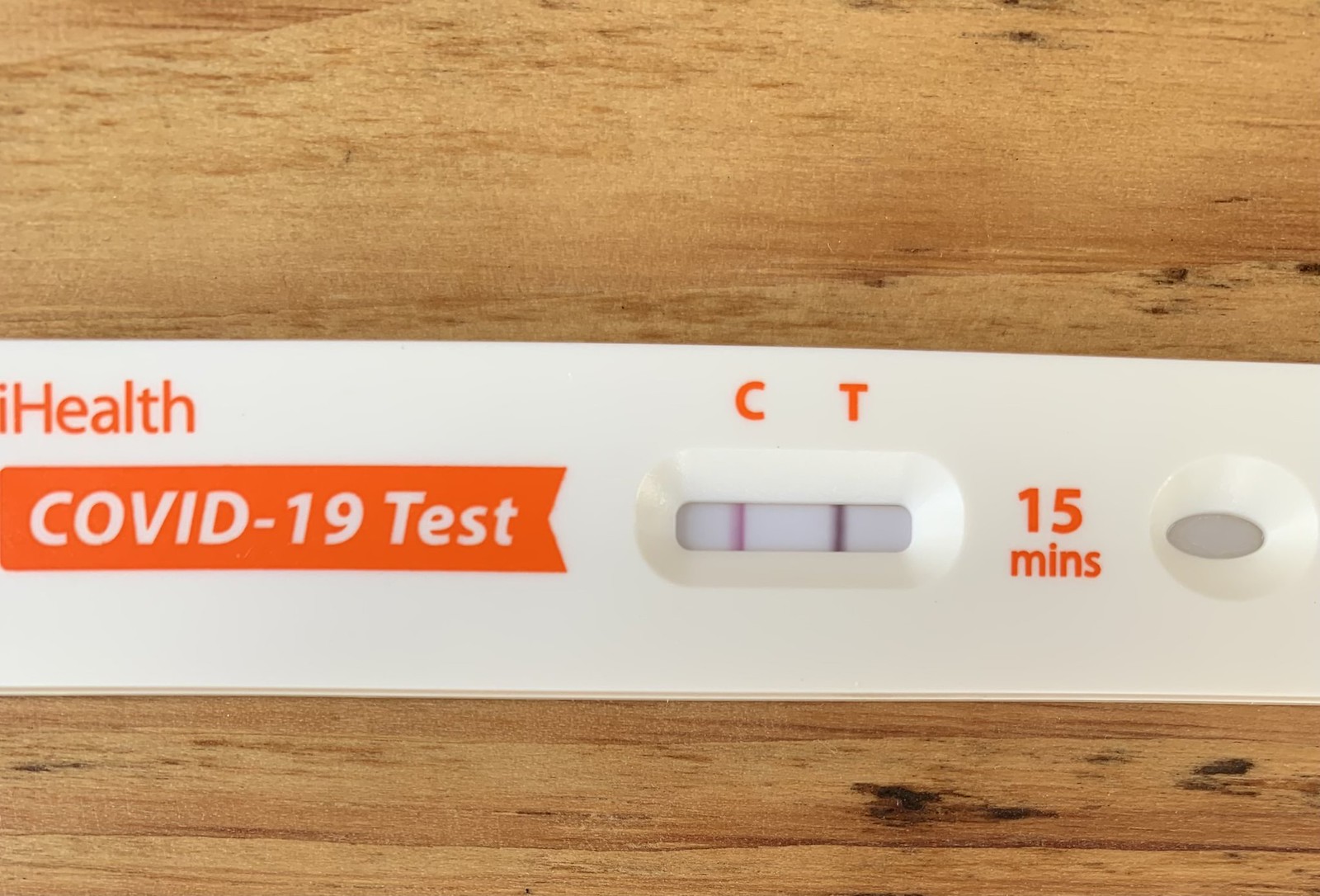A close-up photograph showcases an at-home COVID-19 test kit positioned on an indeterminate wooden surface. The focal point of the image is the white test strip prominently featured against the backdrop. In the upper left corner, partially obscured yellow letters spell out a fragment of the brand name, "Health." 

The test strip itself is marked with crucial indicators labeled with "C" and "T" above the respective result windows. Each window displays a line: a reddish one under "C" and a blackish one under "T," signifying the test's current result status. Above these indicators, the words "15 minutes" are printed in orange. Adjacent to this region sits a circular application area.

The left border of the test strip bears the label "COVID-19 test" printed in white on an orange band, which tapers to a point at the end, giving the impression of an elongated rectangle. The photograph, taken in close proximity, provides substantial detail of the test kit while leaving the surrounding context somewhat ambiguous.